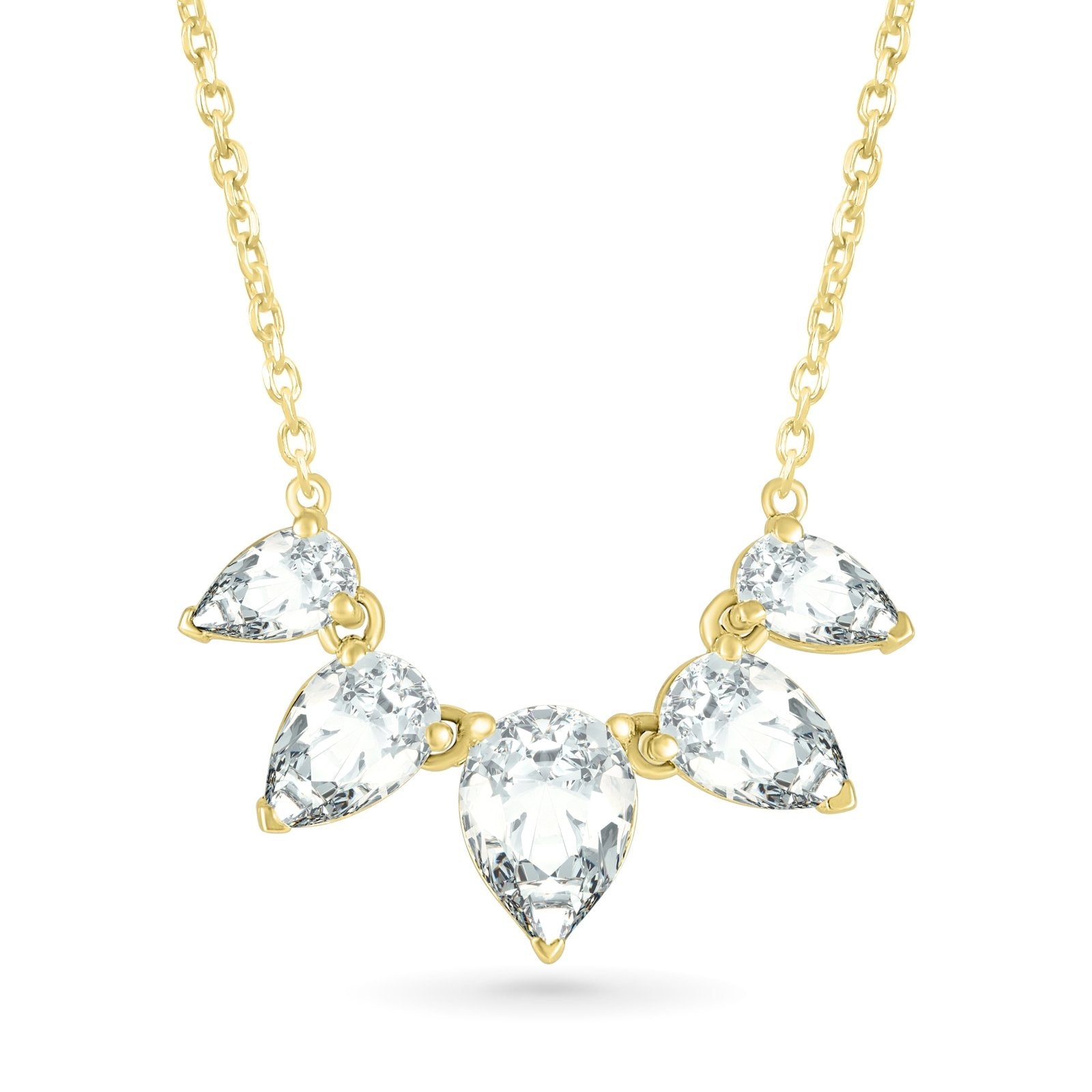This image features a stunning necklace set against a white background. The piece showcases a gold chain constructed from interlinked circular or oval loops. At the forefront, the necklace is adorned with five clear, shiny gemstones, potentially diamonds, cubic zirconia, or similar gems. The gemstones are arranged in an elegant graduated design, with the centrally placed gem being the largest. Flanking the center gem are two medium-sized gems, and at the ends, two smaller ones, all arranged in an upside-down teardrop shape. Each gemstone is accented with a gold tip that points downward, enhancing its refined appearance. This exquisite piece exudes both beauty and sophistication, suggestive of high-quality costume jewelry.